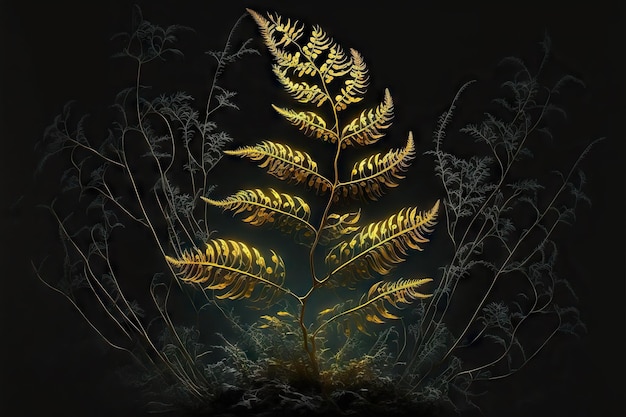The image depicts a color illustration of various plant life, against a dark background with a greenish tinge in the center. The focal point is a vibrant yellow-gold plant, possibly a fern, situated centrally. This plant has teardrop-shaped, detailed leaves and numerous stems. It is widest at the base and tapers off to a point that leans leftward. Surrounding this central plant are more muted, green plants with thinner, arcing stems, creating a sense of depth and contrast. The background plants appear branchy with sparse leaves and minor greenery at the base, suggesting an illustration of growth amidst darkness. The entire composition is both detailed and visually striking, with the golden central plant illuminated to stand out against the darker, subdued surrounding foliage.